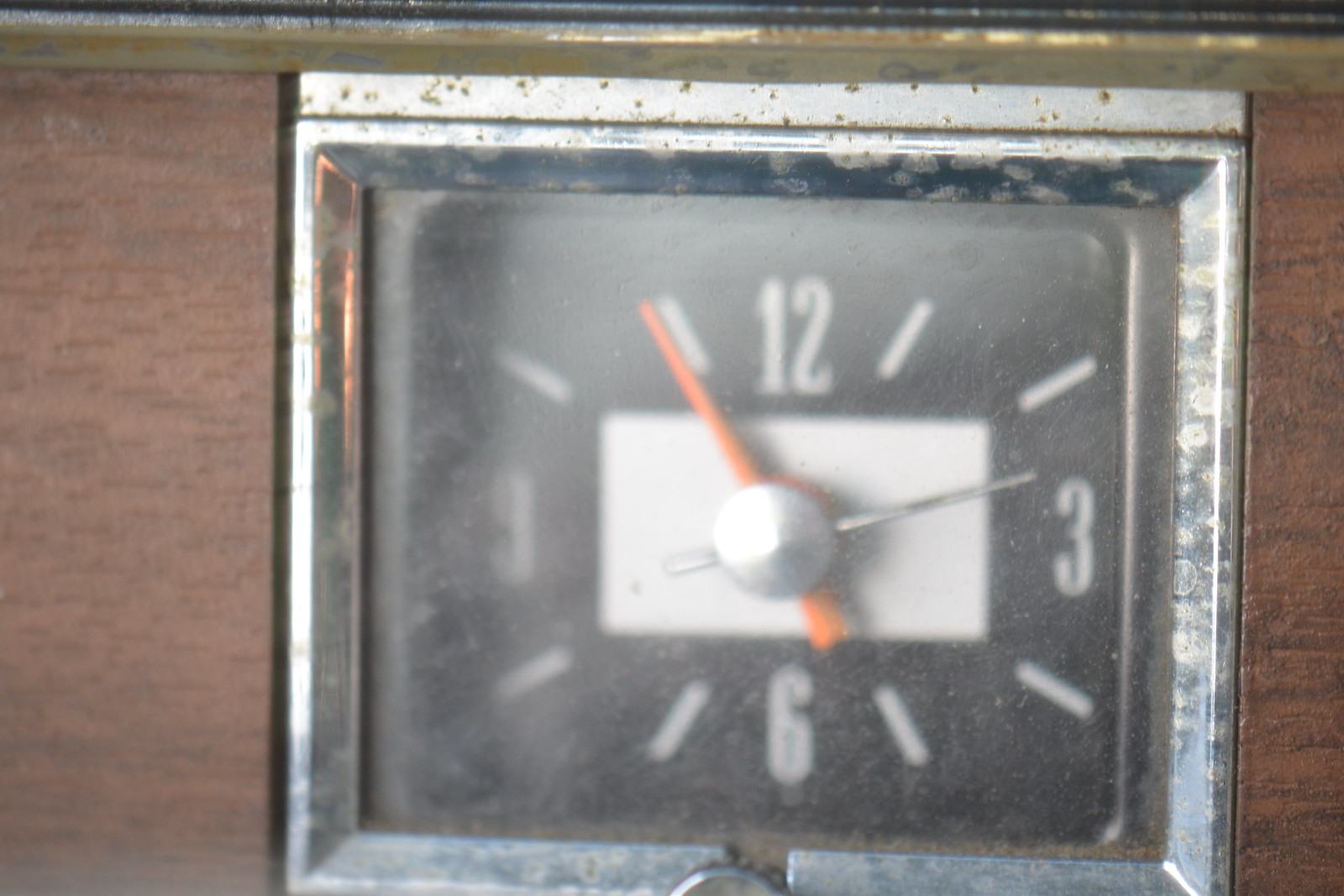An ancient clock nestles within a weathered wooden frame, embodying the essence of timelessness. The clock's metal casing is heavily pitted and corroded, with a once-chrome finish now dulled and battered by the passage of years. Its crystal face, marred by layers of grime, suggests a long period of neglect. The clock face displays the numbers 12, 3, 6, and 9, while the remaining hours are denoted by simple slashes. A white rectangular background offsets the clock's almost rectangular shape. The time is indicated by two striking orange hands, accompanied by a second hand, which may no longer tick. The overall appearance suggests it has been abandoned in a garage for a long time, subjected to the elements and time, casting doubt on its operational status.